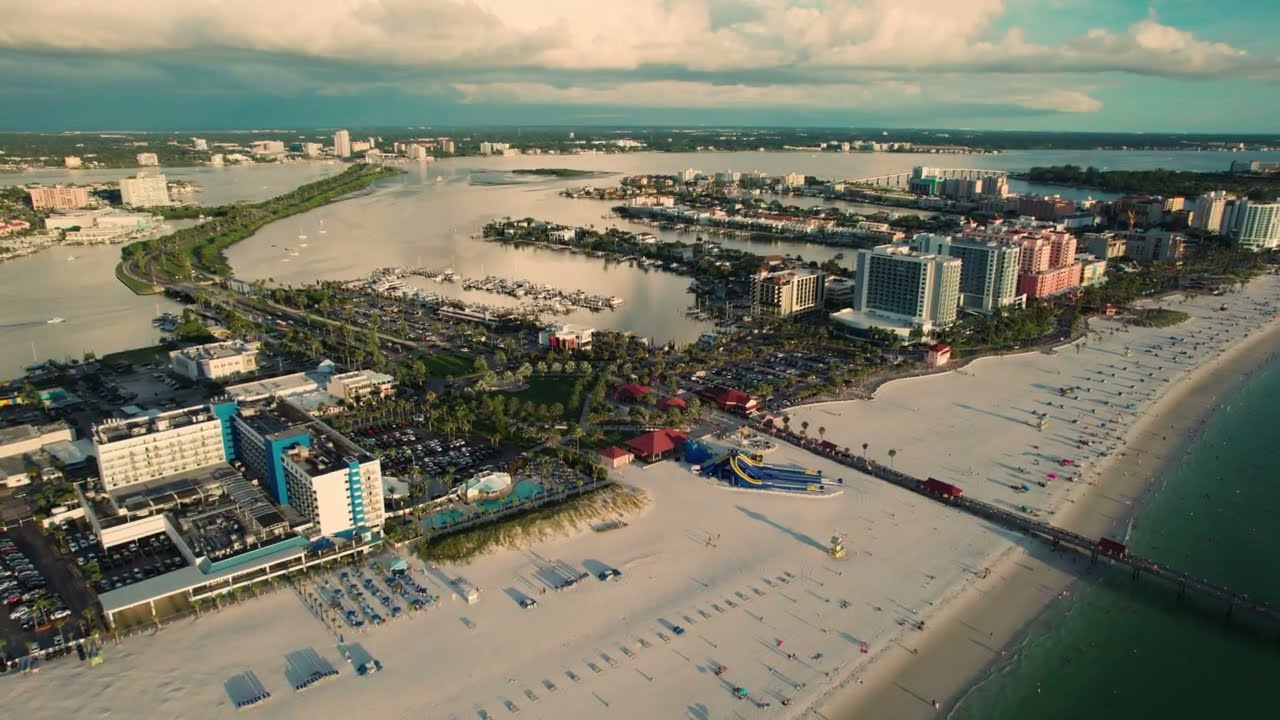This image depicts a vintage-inspired beach resort scene, likely reminiscent of the 1970s, with a slightly darker, nostalgic tone. The camera captures the view from a significant elevation, approximately 100 to 150 feet above the beach, angled gently downward. In the background, a vast expanse of blue water meets a soft blue sky filled with thick, white clouds. A road lined with greenery cuts through the water, leading toward several buildings that appear to be part of a development in the middle of the water and a stretch of what seems to be condos and hotels.

The shoreline features a wide sandy beach extending to the right, bordered by water on either side. This area could be described as a low-lying sandbar, with light-colored sand and a pier jutting out into the darker green waters. The beach itself appears populated with numerous small objects, possibly people and beach accessories, though details are indistinguishable due to the height from which the photo was taken.

Among the buildings, a few skyscraper-like structures dominate the central area of the image, including light green and nearly pink-colored edifices. Smaller buildings populate the surrounding area, with one prominent teal and white structure to the left. Lush plants and greenery are visible along the roads and causeways, enhancing the overall scenic charm of this seemingly idyllic and somewhat isolated beach resort.